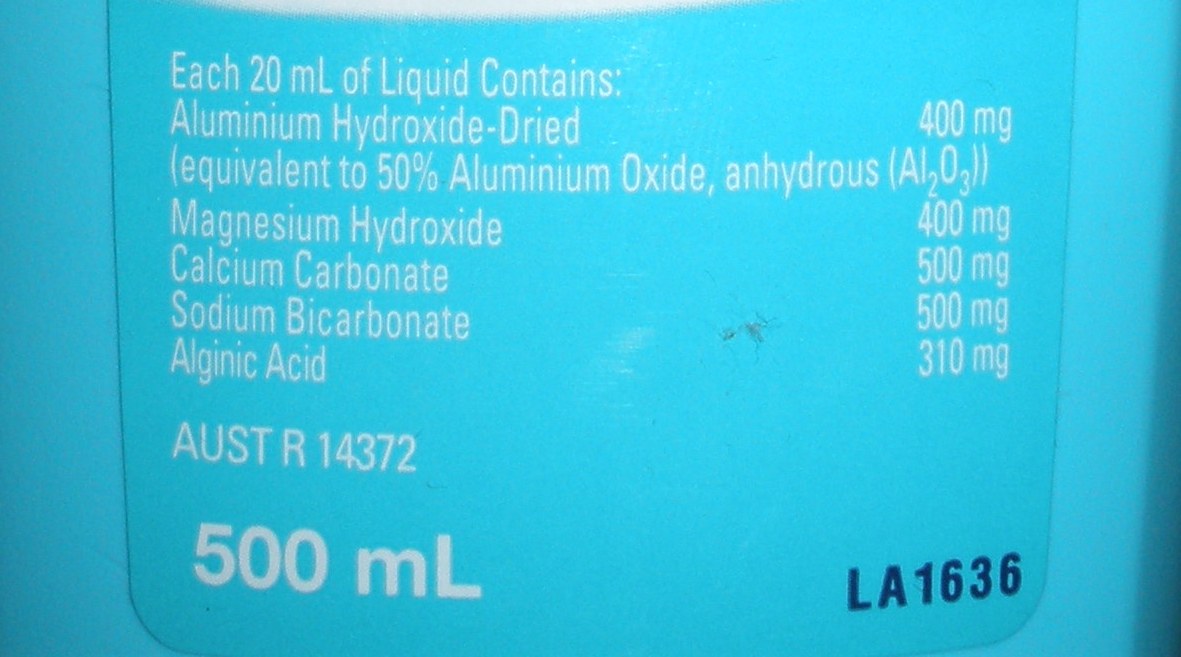The image showcases a close-up view of the back of a blue plastic bottle. The main focus is on the label, which dominates the center of the image, surrounded by slight glimpses of the bottle's curved blue sides. The label details the active ingredients and their quantities. At the top of the label, it reads: "Each 20 ml of liquid contains:". Below this, a list of ingredients is provided along with their respective amounts:

- Alumina Hydroxide Derived: 400 mg
- Magnesium Hydroxide: 400 mg
- Calcium Carbonate: 500 mg
- Sodium Bicarbonate: 500 mg
- Alginic Acid: 310 mg

The detailed listing of ingredients and their precise measurements suggest that the bottle likely contains a liquid formulation for medical or health purposes.